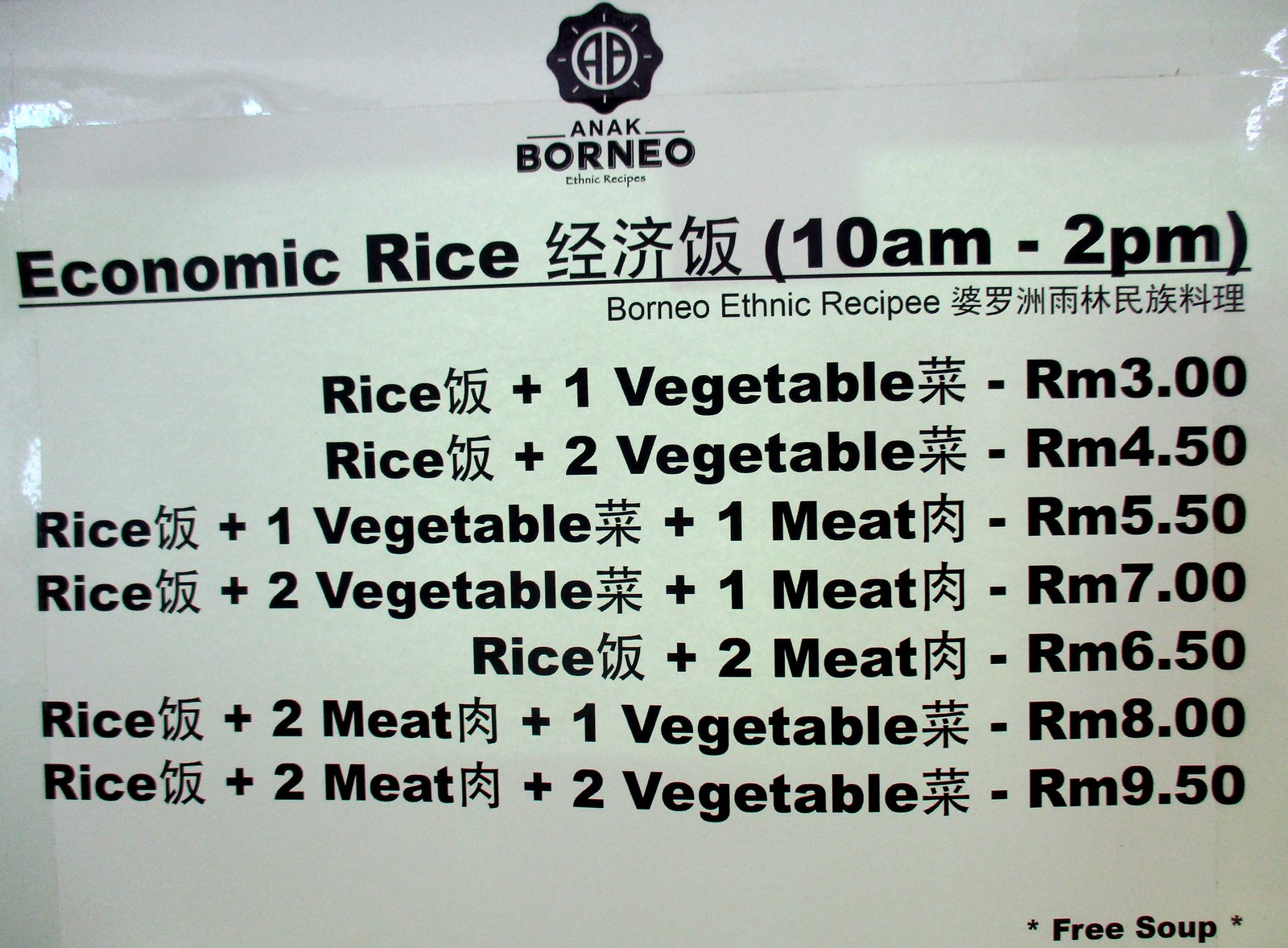This flyer, possibly for a Chinese or Thai restaurant, is printed on greenish-gray paper and prominently features a symbol at the top displaying the letters "AB" encircled, indicating "Anak Borneo" in English. Below the symbol, the text "Economic Rice" is presented alongside some Asian characters, followed by the times "10 a.m. to 2 p.m." The heading "Borneo Ethnic Recipe" is also included. The flyer outlines various meal options, with a detailed menu listing:

- Rice plus one vegetable: RM 3.00
- Rice plus two vegetables: RM 4.50
- Rice plus one vegetable and one meat: RM 5.50
- Rice plus two vegetables and one meat: RM 7.00
- Rice plus two meats: RM 6.50
- Rice plus two meats and one vegetable: RM 8.00
- Rice plus two meats and two vegetables: RM 9.50

In the bottom right corner, an asterisk denotes that free soup is included.